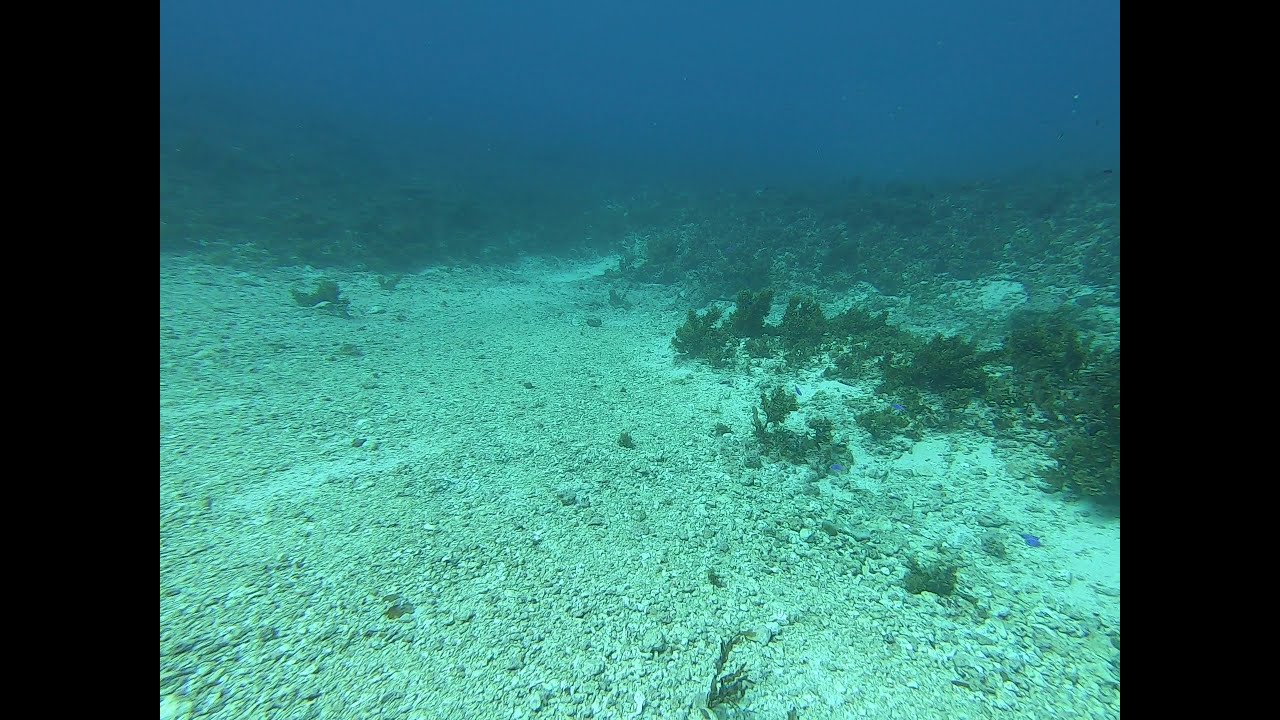The image depicts a dimly-lit, rocky terrain that could either be underwater or a desert landscape at dusk. It is rectangular, with black vertical columns on both sides, framing the central image that is approximately one and a half times as wide as it is tall. The foreground is dominated by small, white rocks mixed with sandy gravel, which appears greenish-gray. Sparse, short green plants are clustered mostly towards the right half of the view, forming a triangular pattern as they extend towards the middle. The upper portion of the image features an indistinct horizon, with rolling hills or mounds covered in green shrubs. The sky or water backdrop is a hazy, dark blue-purple, contributing to the overall low visibility and atmospheric uncertainty about whether the scene is terrestrial or aquatic.